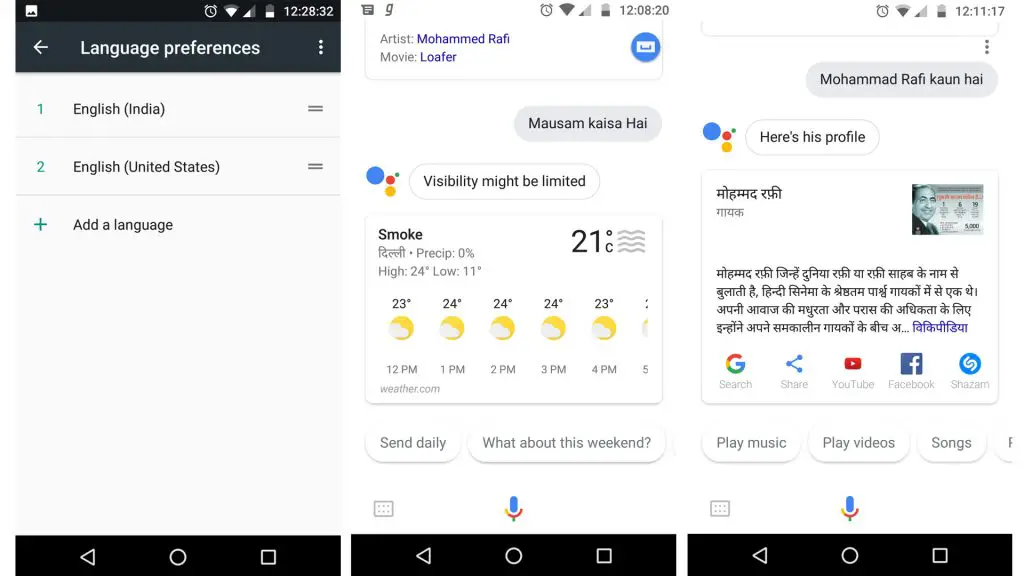The image comprises three separate screenshots from an Android device, highlighting various functionalities of Google Assistant and the device's interface.

1. **Screenshot One (12:28:32)**:
   - **Top Bar**: Displays the status icons from left to right: image icon, timer, Wi-Fi (mostly full), cellular signal (about half), and battery (less than half full).
   - **Time**: 12:28 and 32 seconds.
   - **Content**: Shows an arrow pointing to the left indicating navigation, labeled "Language Preferences" with vertical dots suggesting additional settings.
   - **Languages**: Listed preferences are "1. English (India)", "2. English (United States)", and an option to add another language (+ Add a language).

2. **Screenshot Two (12:08:20)**:
   - **Music Playing**: Features details of the song "M-A-U-S-A-M-K-A-I-S-A-H-A-I" by Mohammed Rafi from the movie "Loafer".
   - **Interaction with Google Assistant**: The user queries in Hindi, and the response shows weather information: "Visibility might be limited", with a Celsius forecast (High of 24°C, Low of 11°C) covering from 12 PM to 4 PM.
   - **Source and Options**: Weather information sourced from weather.com, with options to "Send daily" updates or "Ask about this weekend".

3. **Screenshot Three (12:11:17)**:
   - **Second Song Query**: The song "K-A-U-N-H-A-I" by Mohammed Rafi.
   - **Google Assistant's Response**: Provides details from a Wikipedia-like profile of Mohammed Rafi in Hindi, with various action options.
   - **Additional Options**: Includes actions like "Google Search", "Share", "YouTube", "Facebook", "Shazam", "Play music", "Play videos", and "Play songs".

This series of screenshots effectively demonstrates Google Assistant's language support capabilities and various functionalities, such as language preferences, weather forecasts in different languages, and accessing detailed information about artists and songs with action options.